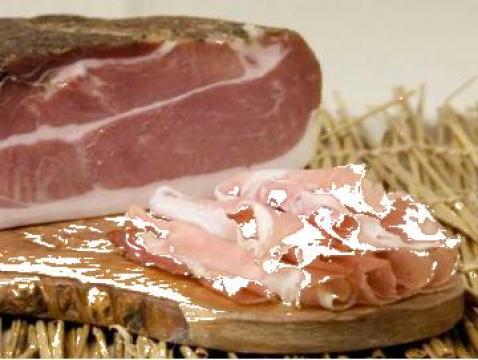The image is a very zoomed-in, slightly distorted color photograph featuring a collection of meats displayed on a wooden cutting board resting on a mat of dried grasses or hay. The main focus is on a glazed piece of ham located in the center-right, which has a sticky, shiny appearance and is laid on top of the wooden board. Thin slices of ham or bacon are also visible in a pile nearby. In the top left corner of the image, there's a full, uncut joint of ham with brown skin and pink flesh, characterized by white fat lines running horizontally. The entire setting is reminiscent of a deli, with colors dominated by shades of brown, pink, white, gray, and tan. Additionally, some areas of the image exhibit white pixel distortion, particularly around the center and bottom left of the chopping board, contributing to the overall visual noise.